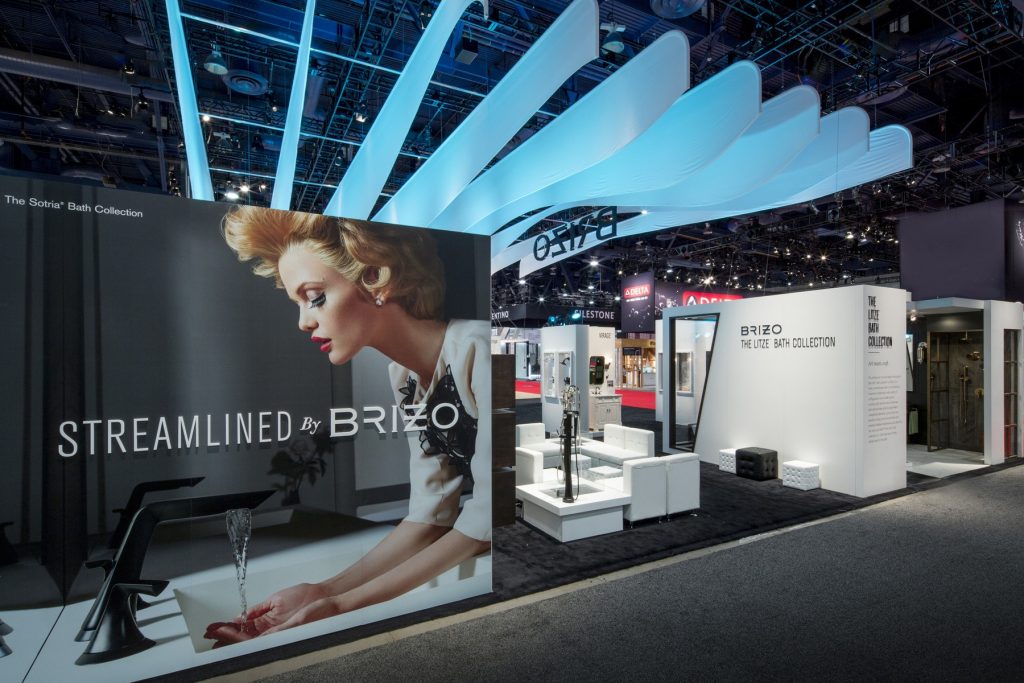In the midst of an expansive, dimly-lit events venue, evidently set before opening hours as no people are present, a striking stand for the Soggia Bath Collection catches the eye. Dominating this booth is a massive, built-in billboard featuring a beautifully stylized graphic of a woman with voluminous, 1950s-inspired blonde curls, her heavily made-up face accentuating her vintage allure. She stands with her arms extended, palms open under a sleek, square sink with modern black taps, water flowing gracefully onto her hands. The setting is sophisticated, with dark greys and blacks contrasting against almost luminous white sheets of material, resembling thin sails, that arch above the stand. Around the Soggia showcase, other booths are discernible but lack detail. The ceiling reveals the venue's structural elements, including overhead lights, metal framework, and ventilation systems, adding to the industrial ambiance. Another neighboring display advertises the Breezo Bath Collection, hinting at a comprehensive bath and kitchen expo filled with sleek, contemporary designs.